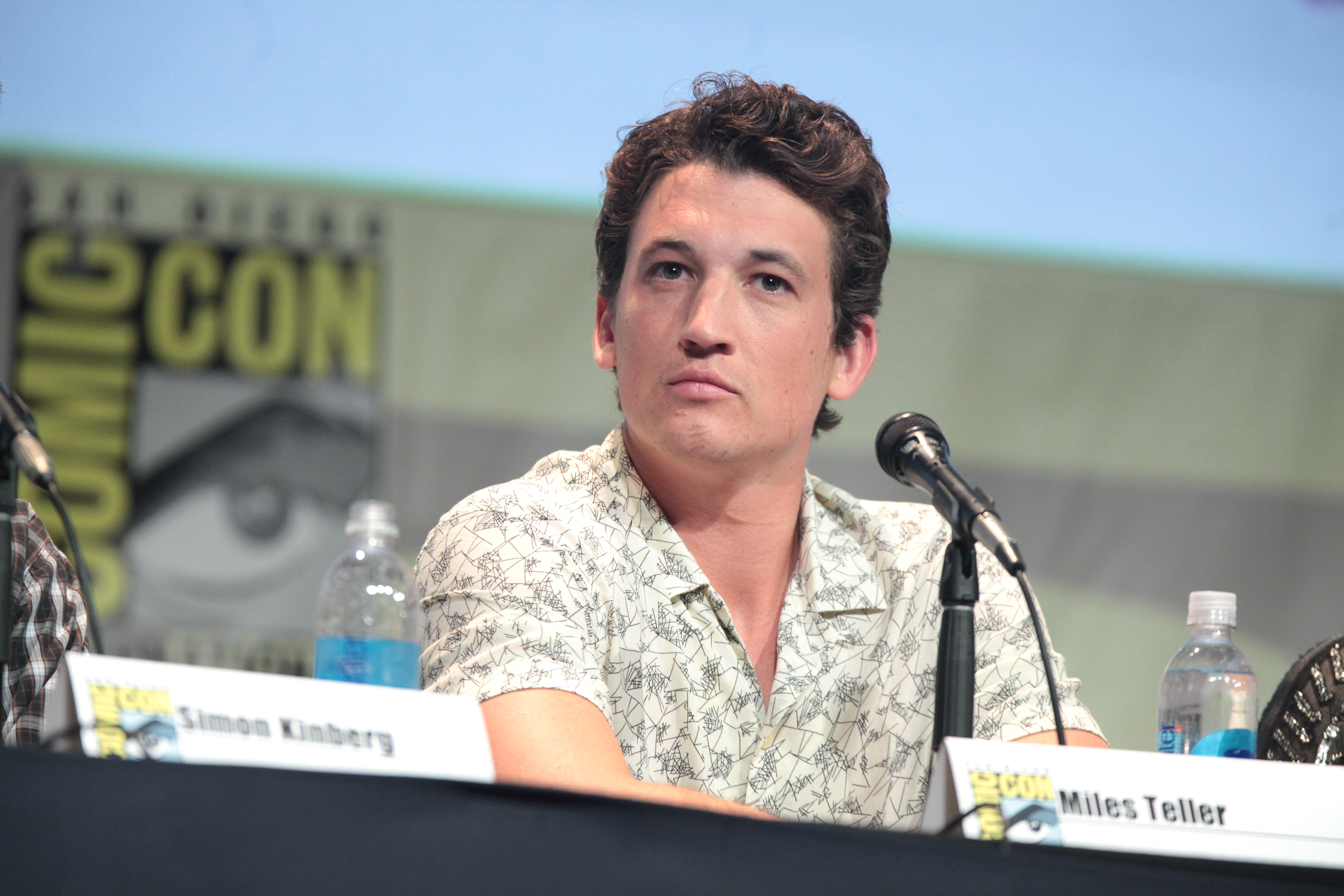The photograph captures a scene at San Diego Comic-Con, featuring a young Caucasian man, likely an actor named Miles Teller, as the central figure. He is seated at a long table draped with a black tablecloth that spans the entire bottom of the image. Miles is positioned almost directly in the center, looking towards the camera with a relaxed yet attentive expression. He has brown slicked-back hair, brown eyes, and is wearing a short-sleeved, button-up shirt with a cream base and black zigzag patterns. 

In front of him lies a white place card displaying his name, "Miles Teller," in black text, accompanied by the Comic-Con logo. Flanking him are two clear water bottles. To his left, partially cropped out, another individual with a brown and white plaid shirt appears, identified by a name tag that reads "Simon Kinberg." Both individuals have black microphones in front of them.

The backdrop sets the scene at Comic-Con, featuring a large sign in black and yellow with the word "Comic-Con," although somewhat blurry. Part of a comic book character's face, particularly the eyes, is also visible in black and white. The background transitions from blue at the top to brown near the center and bottom, suggesting an indoor setting with varied wall surfaces. The atmosphere exudes a lively convention vibe, encapsulated in the Comic-Con setting.